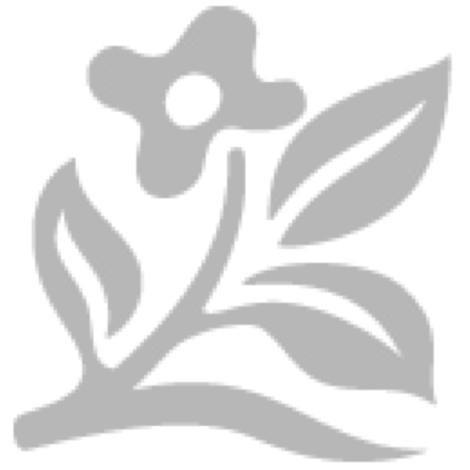The image showcases a striking close-up of a tall, lush burning bush with vibrant, bright red leaves dominating the frame. Numerous slender, long branches extend throughout the plant, each adorned with an abundance of oval-circular leaves approximately an inch long. The leaves exhibit a beautiful gradient, with the upper side radiating a rich red hue and the underside displaying a softer, medium pink shade. In addition to the vibrant foliage, some branches are dotted with small, white flowers resembling popcorn. The background is blurred, revealing hints of green plants, but these are muted and do not detract from the primary focus on the bush's vivid red leaves and dynamic branches.